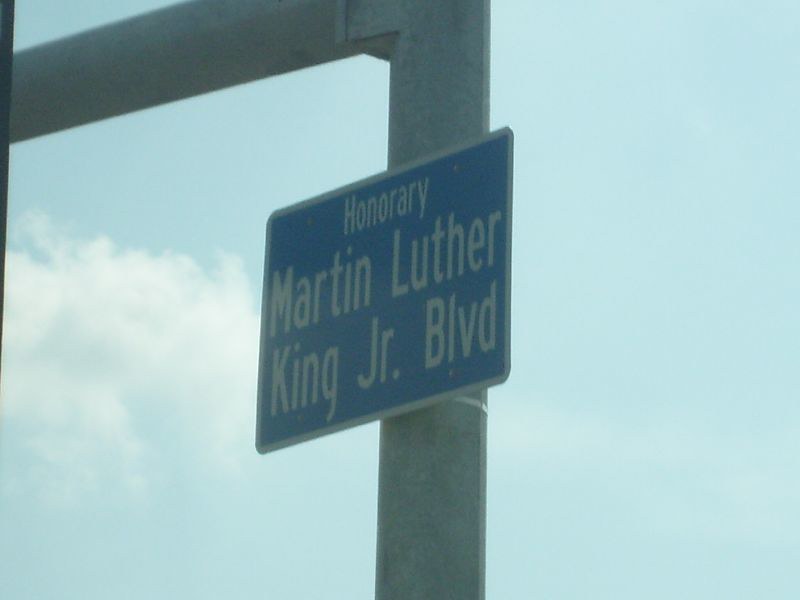This image captures a close-up view of a street sign mounted on a metallic pole. The sign features a blue background with a white frame and is divided into three lines of white, sans serif text. The top row reads "Honorary" in capital letters. The second row, in title case, displays "Martin Luther," with a space separating the two words. The third row, also in title case, spells out "King Jr. Blvd," with appropriate spacing and punctuation.

The sign is affixed to the pole using an L-shaped bracket, visible on the right side of the image. The background showcases a clear daytime sky in light blue, dominated by a large, puffy cloud with wispy edges towards the left. Additionally, a slender, black vertical strip appears on the far left edge of the photograph, potentially the edge of another object inadvertently captured in the frame.